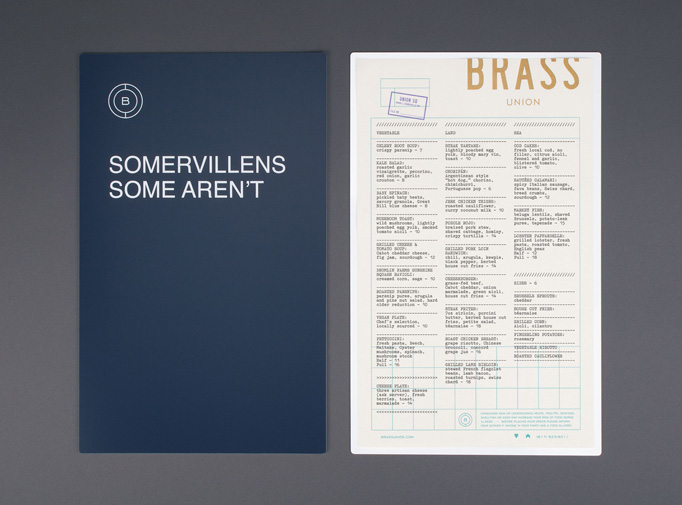The image depicts a detailed visual illustration of a navy blue portfolio cover with white text that creatively plays on the words "summer villains," reading as "some are villains, some aren't." The cover features a distinct logo of a letter "B" encircled in the upper left corner. The background has a slightly grainy, dark gray texture, reminiscent of a desktop surface. To the right, an inside page of the portfolio is visible, featuring a creamish background with text arranged in three columns. The top of this page prominently displays the words "Brass Union" in large, green letters. A teal grid pattern adorns the bottom of the page, alongside another logo. The overall arrangement is well-curated and officially designed, giving an impression of professionalism and attention to detail.